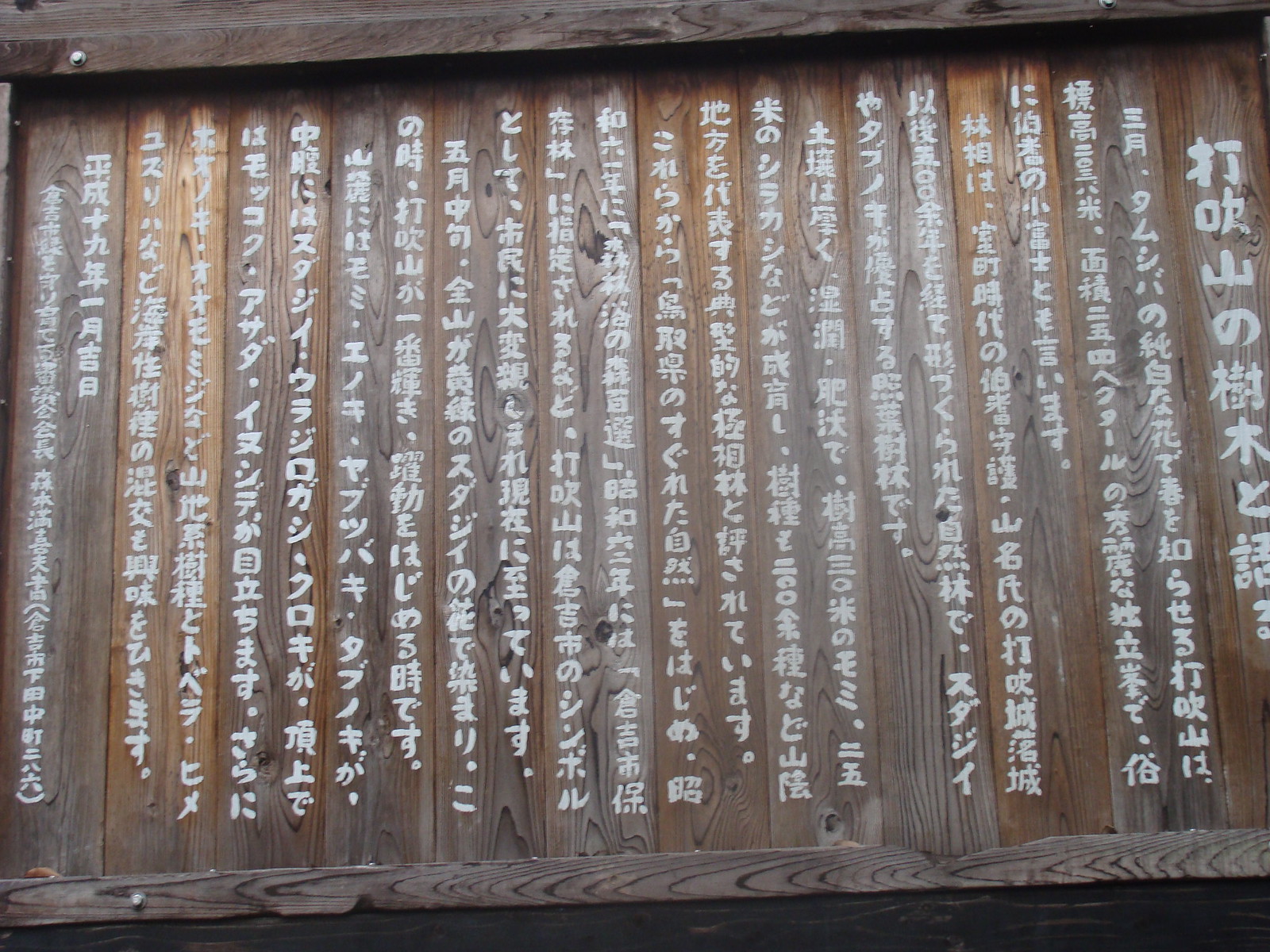This is a rectangular horizontal image of a wooden board featuring vertical Japanese characters. The board is attached to a wall, visible by the presence of nails or bolts. The writing spans across 10 vertical wooden boards, each containing two columns of characters, making a total of 20 lines of text. The characters are written in white and are vertically oriented. Two elongated wooden sections frame the central boards at the top and bottom, protruding slightly further outward. The top left, top right, and bottom left corners of these elongated sections are secured with bolts, while the bottom right is bolt-free. On the far right and far left of the central section, there are larger and more distinct characters that might indicate titles or significant annotations.